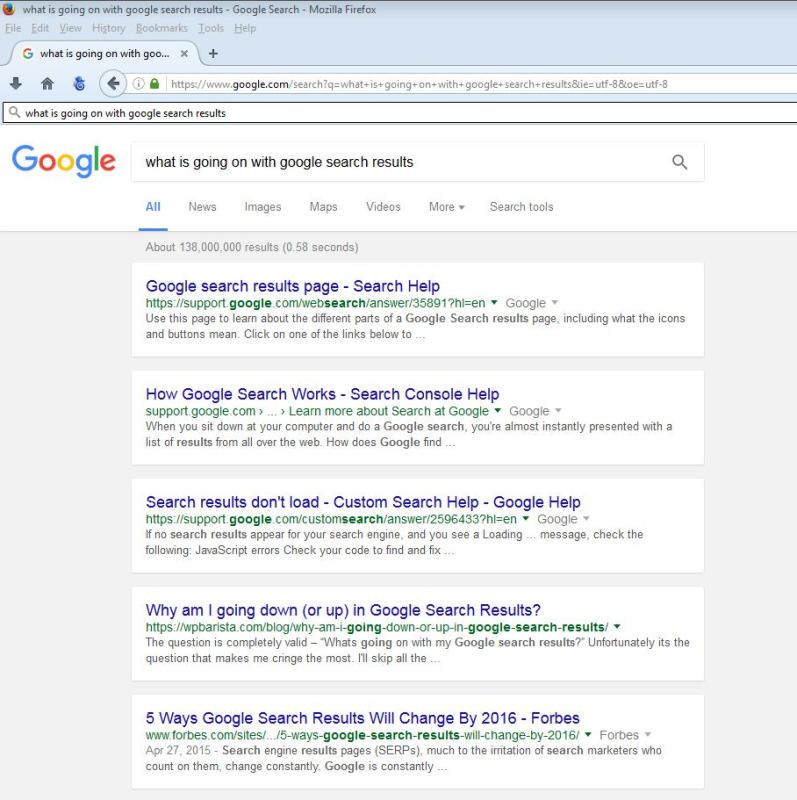A detailed screenshot of a Google Chrome page displays a typical browser interface. This includes an address bar and navigation buttons such as back, home, and refresh located at the top. The browser's menu bar lists options for File, Edit, View, History, Bookmarks, Tools, and Help from left to right.

At the very top, next to the Google Chrome icon, the page's tab reads: "What is going on with Google search results - Google Search - Mozilla Firefox." Below the address bar, a search field is filled with the query "What is going on with Google search results?"

Just beneath this, another search bar from Google displays the same query. Under this search bar, there are menu options for refining searches, including All, News, Images, Maps, Videos, More, and Search Tools. A message indicates approximately 138 million results were found in 0.58 seconds.

The first search result is titled "Google Search Results Page - Search Help." Following this, the second result is "How Google Search Works - Search Console Help." The third result reads, "Search Results Don't Load - Custom Search Help - Google Help." The fourth result asks, "Why Am I Going Down or Up in Google Search Results?," and the fifth result is "Five Ways Google Search Results Will Change by 2016 - Forbes."